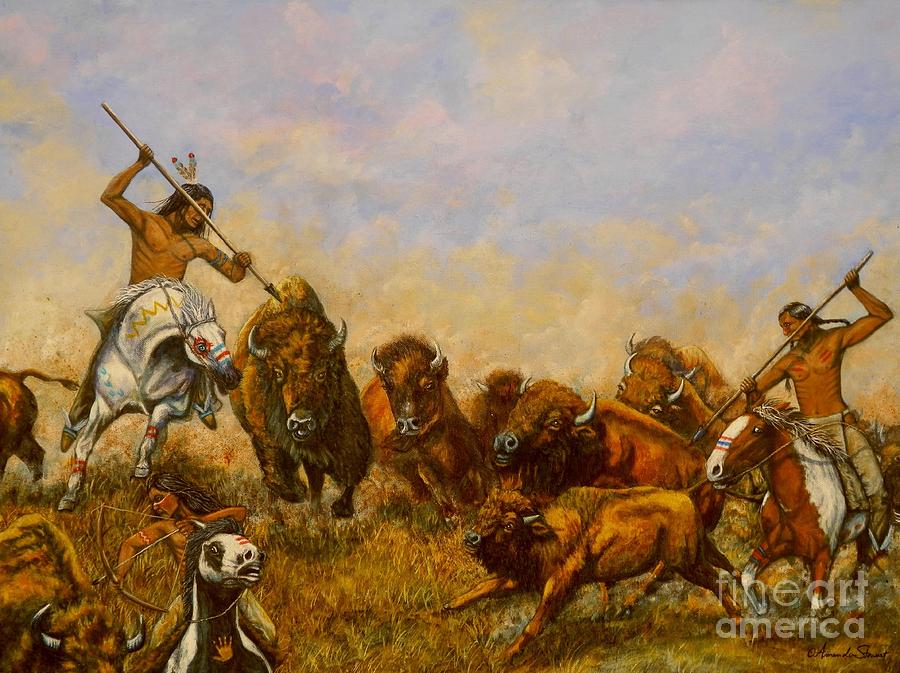This detailed painting captures an intense outdoor scene of Indigenous people hunting buffalo. Central to the composition is a herd of brown buffalo with prominent horns and large humps, running forward. At the bottom right corner, the ghosted text "Fine Art America" appears over a faint image of horns.

On the right side of the painting, an Indigenous man with black hair in a ponytail and red stripes on his chest is prominently shown. He is shirtless and thrusts a spear into the back of one of the buffalo. On the far left, another Indigenous man is mounted on a white horse adorned with a blue and red stripe across its nose. He also holds a spear, aimed at a buffalo. In the bottom left corner, a third Indigenous man is depicted riding a black and white horse with a distinctive brown paw print on its chest. This hunter is in the act of shooting a bow and arrow at the buffalo.

The scene is rich with colors including shades of brown, gold, light blue, off-white, tan, black, red, and blue, evocative of an outdoor, daytime setting. The painting effectively captures the dynamic movement and historical context of a buffalo hunt, immersing the viewer in the vibrant and pivotal moments of the hunt.